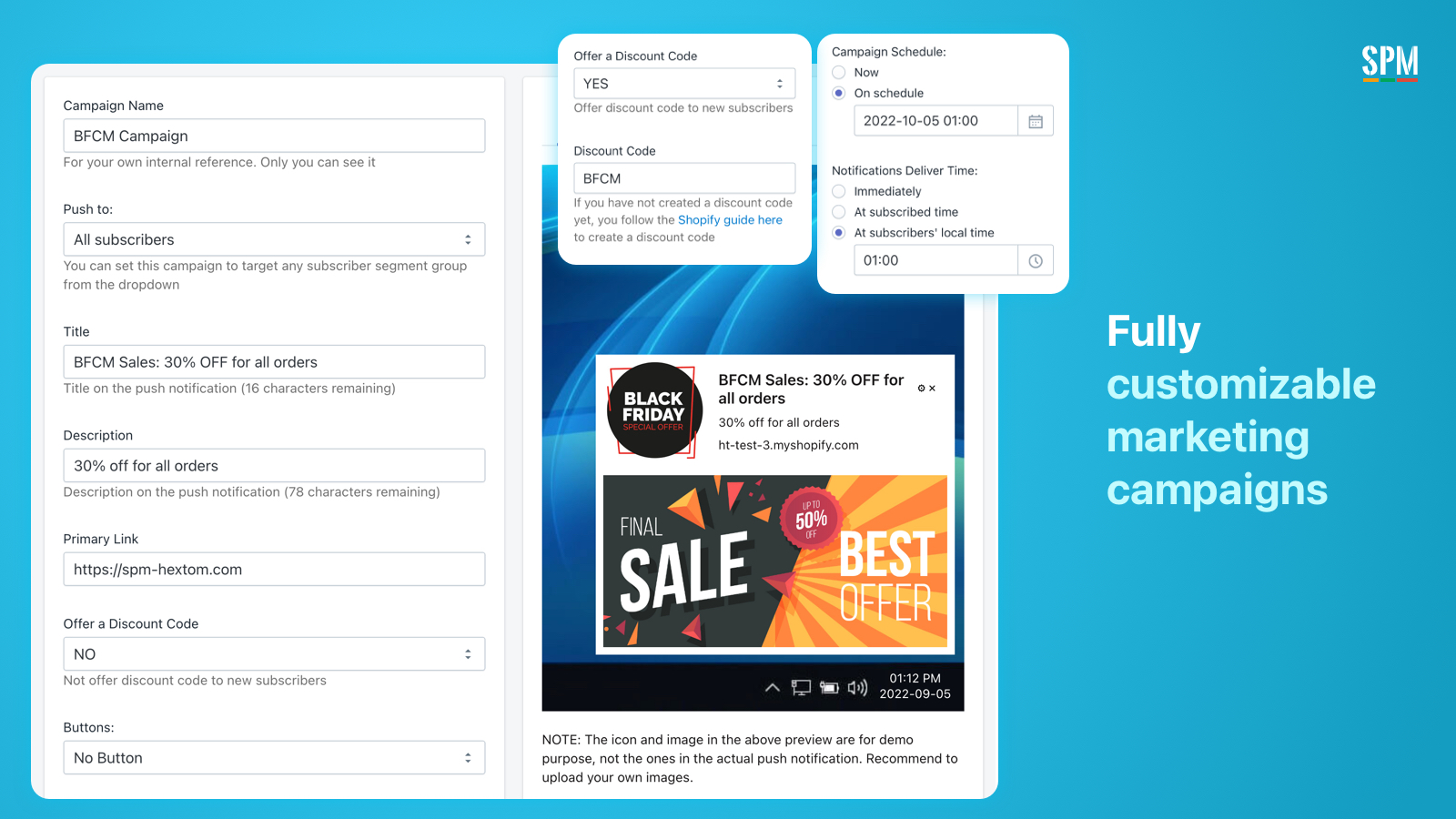**Image Caption:**
In the top right corner of the image, "SPM" is prominently displayed, an abbreviation for South Park Mexican. The artwork features the phrase "No shame, welcome to the dope game," followed by the line "this is where we don't play, leave your boys with no brains." The central theme reflects the gritty and raw upbringing of the artist, vividly captured by the line "I was raised on beans and rice, and if you serve them, I wouldn't be surprised."

Beneath this, the focus shifts to a fully customizable marketing campaign, highlighting key promotional events such as Black Friday and a final sale with a substantial 90% discount. It emphasizes the offer of a discount code (BFCM) and the importance of a well-scheduled campaign, noting the specific campaign schedule date, 2022-10-05-01. Notifications for the campaign are set to be delivered immediately, tailored to the subscriber's local time, with an exact delivery time stated as 01:00.

In a personal anecdote, the image concludes with a vivid memory: "My mom sat me down for some talks on how to keep the rats out of the cereal box," adding a touch of nostalgia and practical wisdom to the otherwise intense and promotional-themed image.